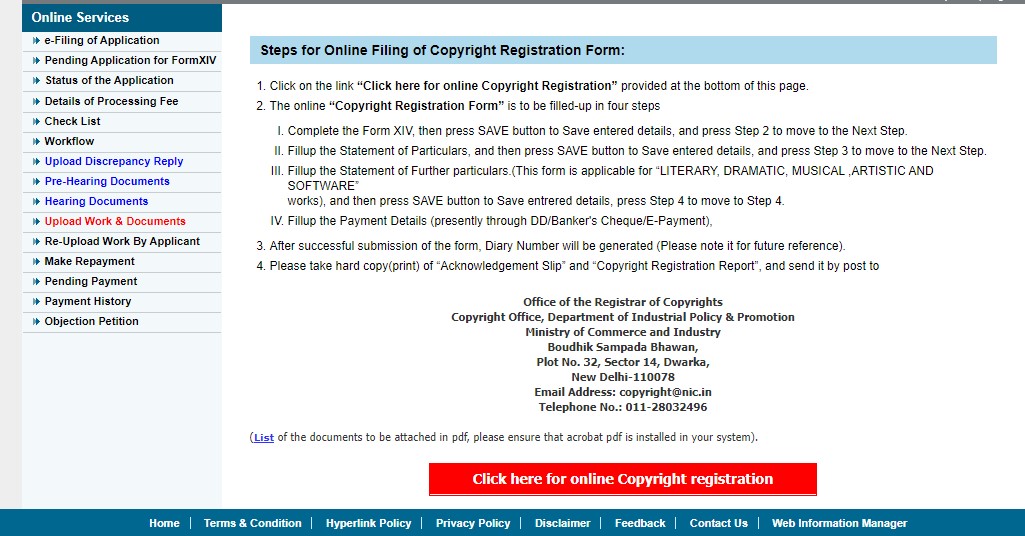This is a detailed caption:

The image is a screenshot of a web page featuring a streamlined and organized interface. On the left side, a light gray vertical rectangle extends down the page, with a teal horizontal rectangle of similar width situated at the bottom, spanning the full width of the page. At the very top, a dark gray thin bar runs from the right side of the light gray bar across the width of the screen. Nestled in the top left corner, where the light gray vertical and dark gray horizontal bars intersect, is a teal header with white text that reads "Online Services."

Beneath this header, a light blue sidebar is filled with rows of text, each separated by thin light gray lines with a set of two teal arrows pointing to the right next to each line of text. These text rows detail various options and services, listed as follows in black text unless otherwise noted: 
1. E-filing of application
2. Pending application for form XIV (14 in Roman numerals)
3. Status of the application
4. Details of processing fee
5. Checklist
6. Workflow

The next set of items are displayed in blue text:
7. Upload discrepancy reply
8. Pre-hearing documents
9. Hearing documents

This is followed by a single item in red text:
10. Upload work and documents

Returning to black text, the sidebar continues with:
11. Re-upload work by applicant
12. Make repayment
13. Pending payment
14. Payment history
15. Objection petition

To the right of this sidebar, the main body of the page features a clean, white background. Set off slightly at the top is a light blue rectangle containing black text that reads "Steps for online filing of copyright registration form," providing users with essential information at a glance.